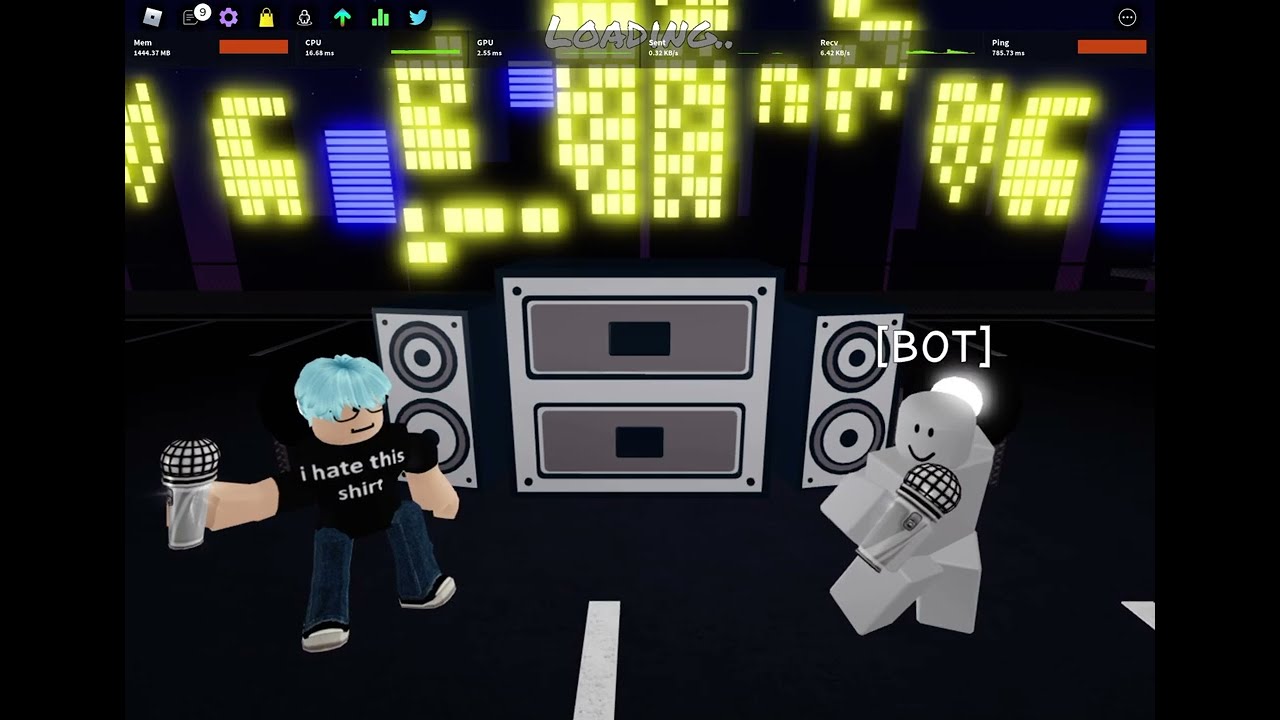In this vibrant animated scene set against a flat black background, two blocky, Lego-like figurines stand on what resembles a black road. On the left, a character with short, straight blue hair, glasses, and Caucasian skin wears a black shirt emblazoned with “I hate this shirt” in white print, paired with dark blue jeans and black-and-white shoes. Holding a silver microphone in his extended right hand, he stands confidently in the foreground. Opposite him, a light gray block figurine with a simplistic smiley face, comprising two black dots for eyes and a black line for a mouth, appears to be dancing while also holding a silver microphone. Between them is a large, silver-gray sound system flanked by two rectangular speakers with round gray speaker rings. Above these figures, block-styled yellow lights illuminate the scene, with blue sound bars adding to the dynamic background. At the top of the image, the word "loading" is prominently displayed, hinting at an interactive or gaming environment.